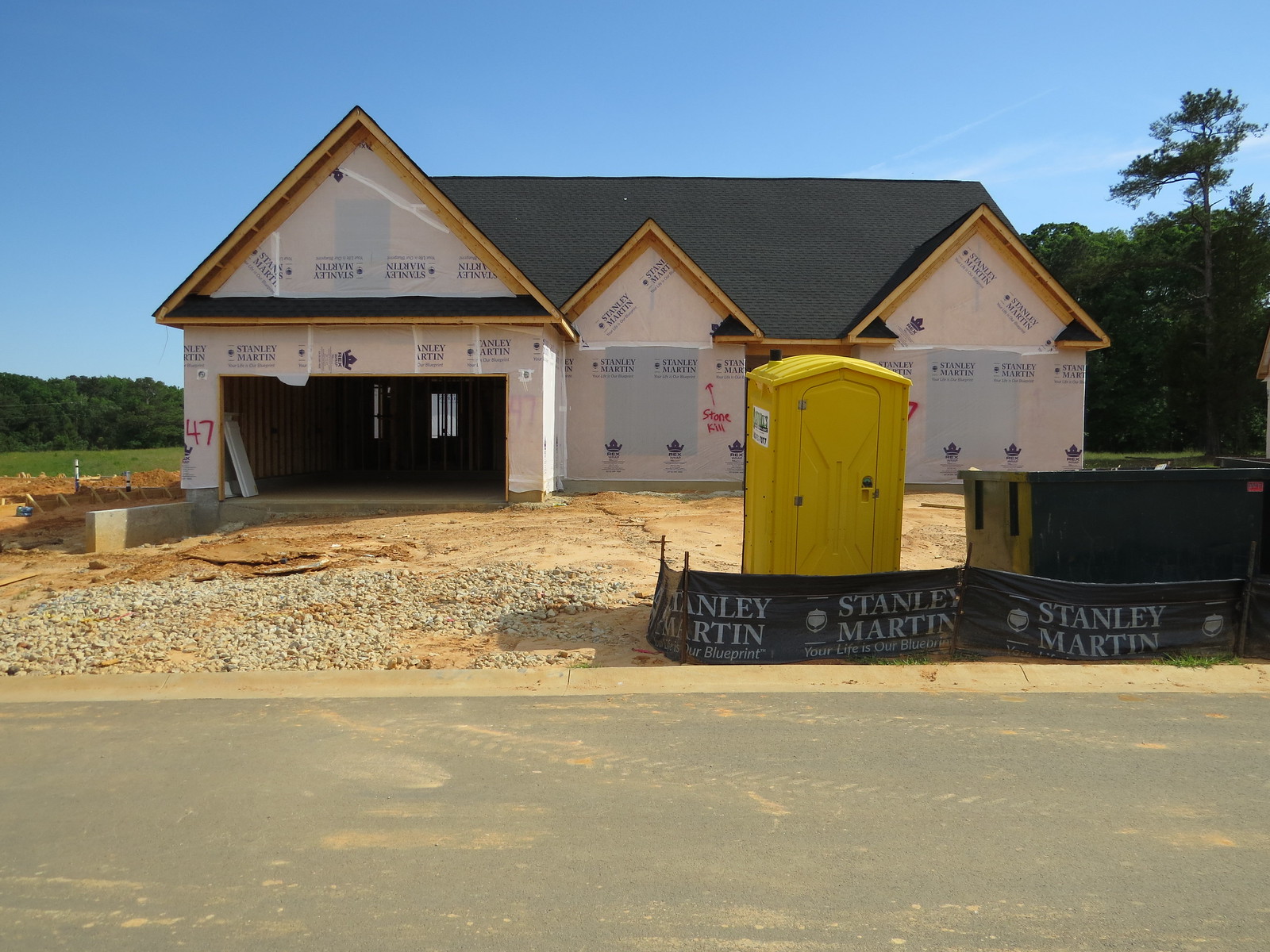In this image, the central focus is an unfinished house located in a working construction site. The house, with its white siding and black roof, features an open door or garage on the left side and some light brown wood accents. Surrounding the house is a concrete gray street occupying the bottom fourth of the image. Directly in front of the house, an unfinished driveway is covered with brown dirt and green or gray gravel. 

To the right of the house, there's a yellow port-a-potty, positioned next to a blue-green dumpster. Both items are bordered by fencing, and a banner on the fence reads, "Stanley Martin, your life is our blueprint." This banner is also noted in front of the yellow structure. There is greenery on both sides of the house, with light green grass and fields to the left and additional trees framing the scene on the right. 

The top background portion showcases a light blue sky, indicating a clear day. The site is adorned with various stickers and the number 47 is visible on the house. An additional sign reading "Stone Hill" with an arrow pointing upwards is seen in red. Overall, the scene provides a detailed depiction of a construction site in progress, with tools, materials, and structures indicative of a future residential area.